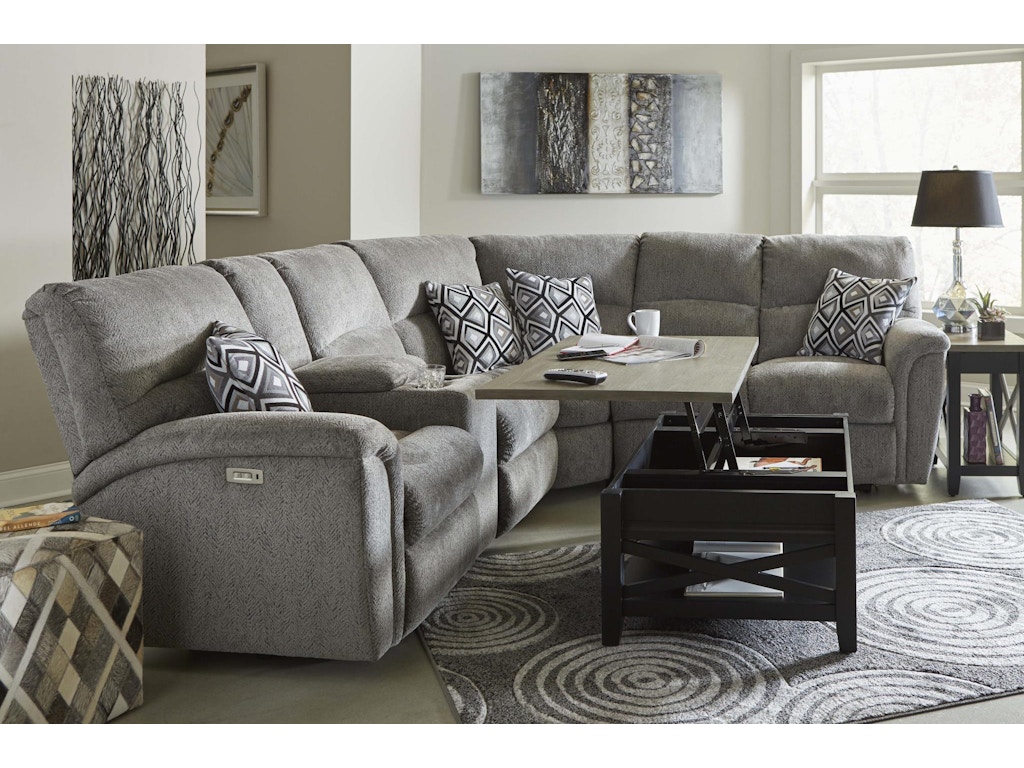This is a detailed image of a modern living room showcasing a contemporary and meticulously arranged interior. The central focus is a gray sectional sofa with built-in powered recliners, evidenced by the visible control buttons on the side. Accompanying the sectional are four geometric-patterned throw pillows in shades of gray, white, and black. The floor features a gray area rug adorned with white concentric circles, contributing to the room’s contemporary aesthetic. 

A standout feature of the room is a multifunctional black coffee table with an off-white or light gray lift-up top. This coffee table, designed for convenience, holds a TV remote, a coffee cup, a magazine, and a pad of paper, indicating it is actively used. Adjacent to the sectional is a side table, topped with a lamp featuring a black lampshade and a small plant.

On the left side of the image rests a tan, gray, and white diamond-patterned ottoman. The walls, painted white, are decorated with abstract canvas artworks in black, white, and gray tones, adding an artistic flair to the space. A large, unobstructed window allows natural light to permeate the room, providing a view of the yard outside. This picture, reminiscent of a stylish furniture advertisement, captures the essence of a clean, contemporary living space in neutral tones.